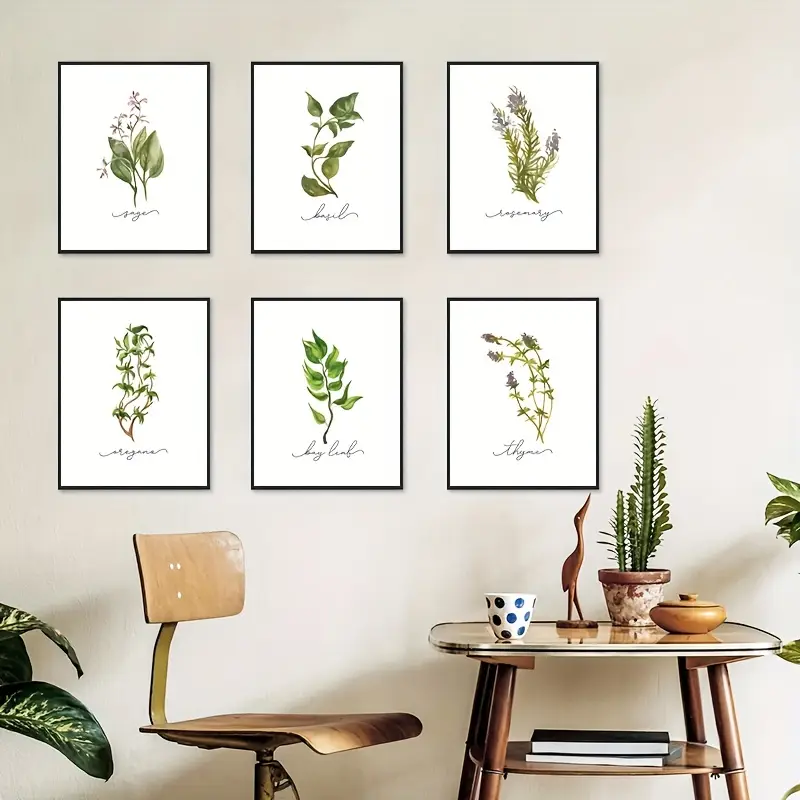This image depicts a cozy, home office nook designed with an art gallery flair. The focal point is a collection of six intricately detailed botanical illustrations, each framed in sleek black frames and arranged in a grid of three by three on a white background. These images, presumably drawn in green pencil, showcase various plant species, likely herbs, adding an artistic touch to the space.

In the foreground, there is a vintage-style wooden chair reminiscent of an old-school classroom seat, with a curved wooden back and a contoured seat. The chair is paired with a table that features four wooden legs and a glass top. This table holds a few carefully selected items: a coffee mug, a small wooden sculpture of a bird, a cactus in a pot, and a wooden bowl with a lid. 

The table also incorporates a lower glass shelf, which houses two books, adding to the room's intellectual atmosphere. Additionally, a plant to the side complements the overall aesthetic, enhancing the space's natural and serene ambiance. The detailed arrangement of these elements creates a harmonious blend of functionality and artistic expression, perfect for enjoying a morning coffee or tea while surrounded by botanical beauty.